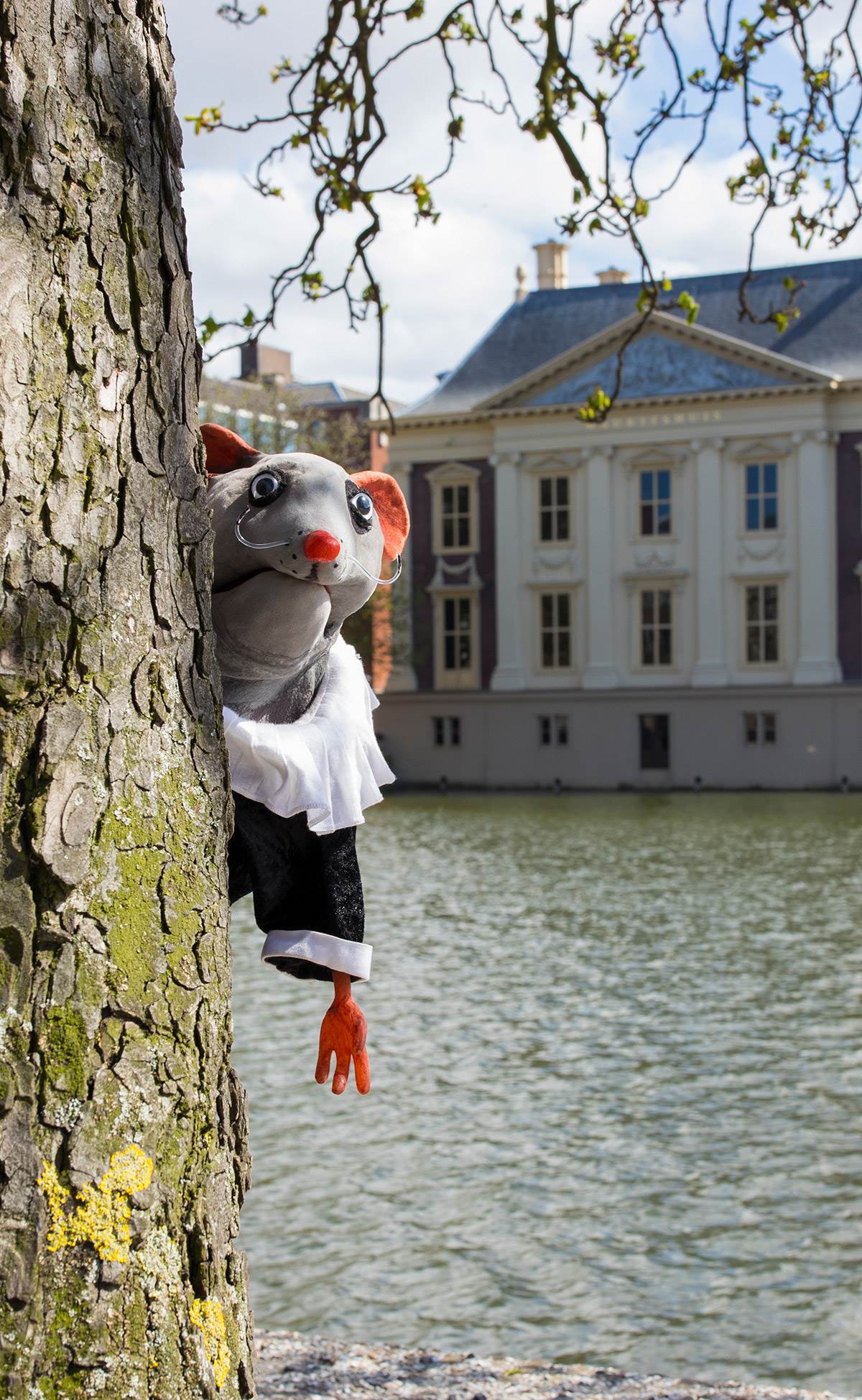In this daytime photograph, a humorous scene unfolds with a large, grey mouse-like character peeking from behind a substantial tree trunk on the left side. The character, garbed in a black and white costume, features orange ears, a red nose with a mustache, and a prominently visible orange hand. The brown tree trunk, adorned with green moss, stands near a green-colored water body resembling a river or stream. In the background, an elegant house with royal architecture, characterized by a blue roof, chimneys, and large windows, is visible. Additional buildings can be seen beyond the house. The clear blue sky, dotted with white clouds, casts daylight across the entire scene, enhancing the vivid colors and playful atmosphere of the image.